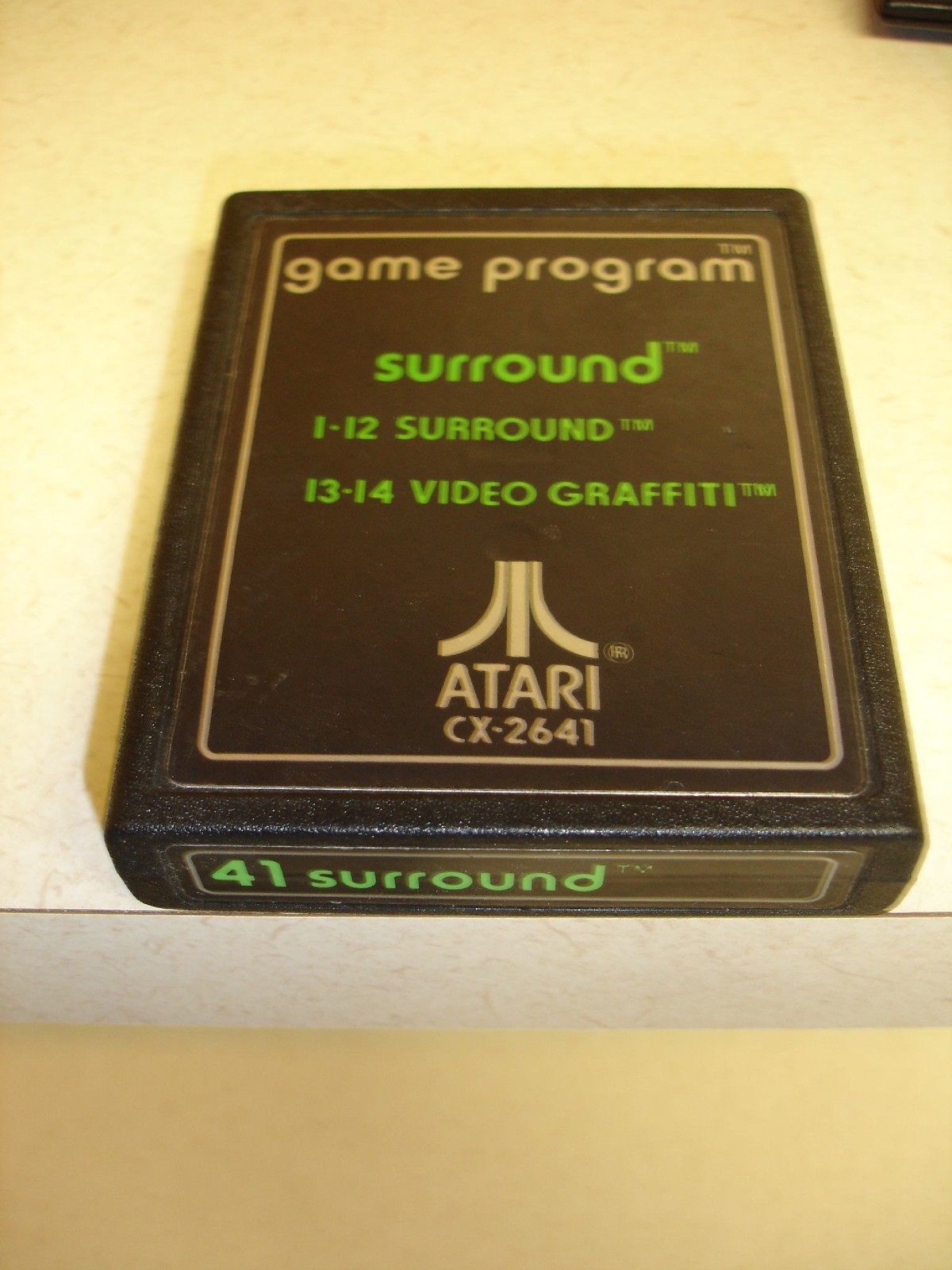The image features a white table bathed in warm, yellow light, creating a yellow hue on its surface and beneath it. Centered prominently on the table is a brown rectangular box labeled "Game Program" in vibrant yellow text. This box appears to be either an old video game cartridge or a storage box for a game-related item. The box's detailed labeling includes "Surround" in green text, followed by "1-12 Surround, 13-14 Video Graffiti". Additionally, a symbol resembling a rocket ship is present, with the model designation "Atari CX-2641" printed below it. The flaps of the box are also visible, and on the bottommost flap, the text "41 Surround" is noted once more. The overall scene captures a nostalgic, vintage item related to the Atari gaming system, invoking memories of retro gaming.